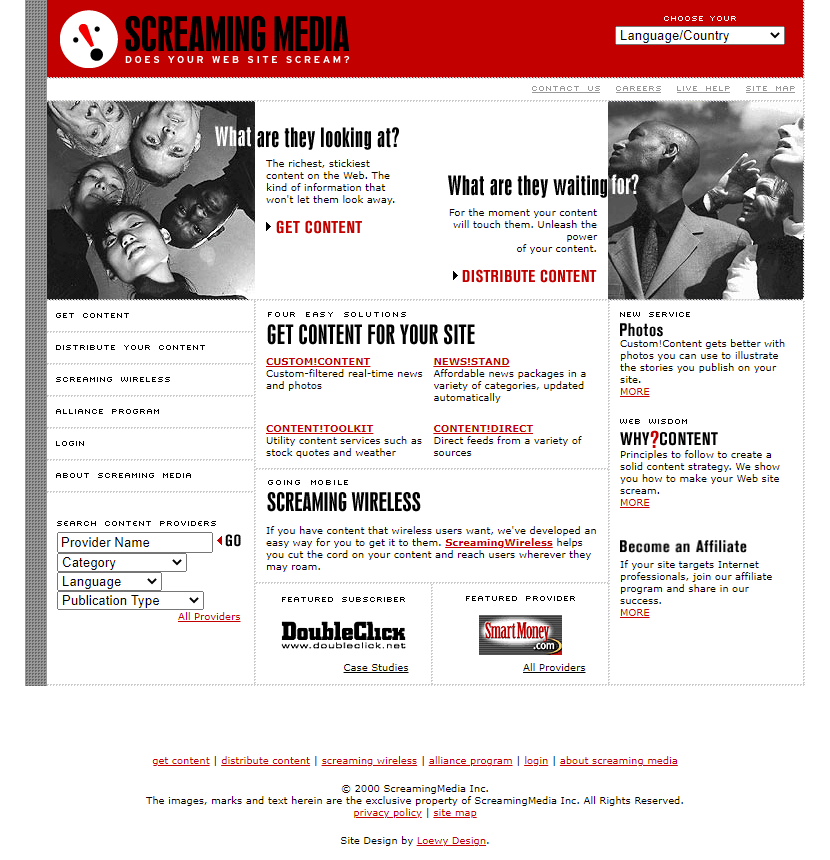This screen capture showcases a web page titled "Screaming Media: Does Your Website Scream?" The top right corner of the red banner provides options to choose your language and country, while the top left corner features a distinctive logo. The logo consists of a white circle paired with three black circles and a red raindrop shape, symbolizing a mouth, nose, and eyes.

Directly below the banner, two black-and-white photos are arranged—one on the left and another on the right. The left photo depicts five men of diverse ages and races, accompanied by the text: "What are they looking at? The richest, stickiest content on the web, the kind of information that won't let them look away. Get content." The right photo shows three different people, also of various ages and races, with the caption: "What are they waiting for? For the moment your content will touch them. Unleash the power of your content. Distribute content."

On the left side of the screen, there is a menu containing the following options: "Get Content," "Distribute Your Content," "Screaming Wireless Alliance Program," "Login," and "About Screaming Media."